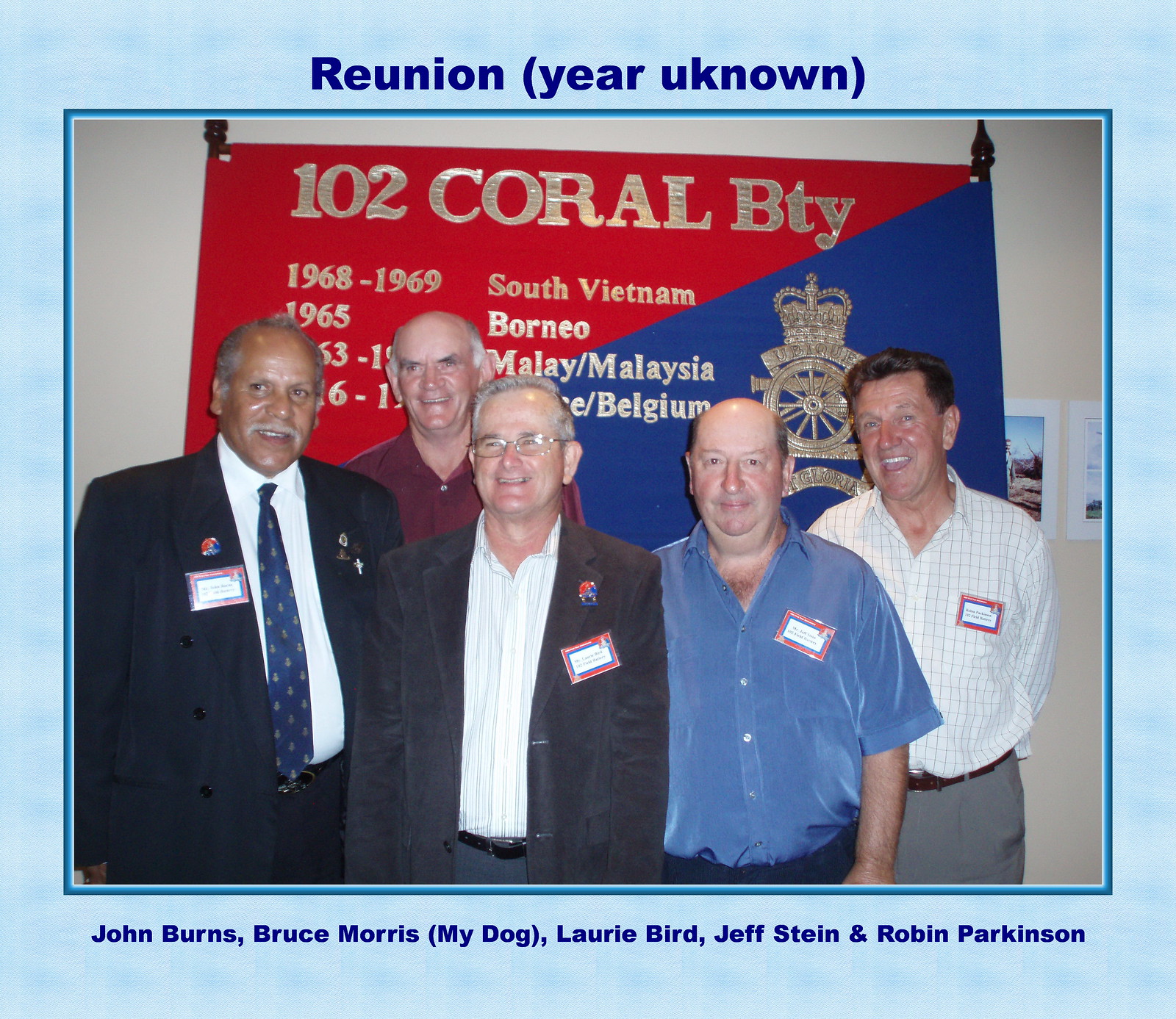In this image, five men are standing shoulder-to-shoulder, appearing to be at a reunion, as indicated by their smiles and camaraderie. From left to right, the first man is an older, heavier African-American with white hair, a mustache, and a business suit complete with a tie and a name tag on his left chest. Next to him stands an older Caucasian male in a red shirt, also smiling but looking slightly off-camera. The third individual, also Caucasian, is dressed in a suit with a white, striped shirt and glasses, similarly gazing away from the camera. The fourth man is wearing a short-sleeved blue shirt and is making direct eye contact with the camera, while the man on the far right, in a striped shirt with square patterns and gray pants, smiles with his mouth open, also looking directly at the camera. Behind them, a red and blue banner forms the backdrop, adorned with various inscriptions such as "BTY, 1968, 1969, South Vietnam," among others. Framing the image is a blue border with text at the top and bottom. At the top, it reads "Reunion, Year Unknown," while the bottom lists the names John Burns, Bruce Morris, Laurie Bird, Jeff Stein, and Robin Parkinson, who are presumably the men in the photograph, indicating that they might be veterans or part of a memorial event.